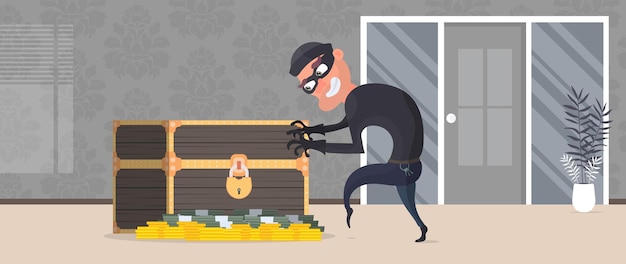A modern cartoon illustration depicts a bandit dressed entirely in black, including a black beanie, black burglar mask, black-rimmed glasses, black gloves, a black long-sleeved shirt, black jeans, and black shoes. Details even show a key ring on his waist and brown eyebrows peeking through his mask. With a big smile on his face, revealing his teeth, he is crouched over, doing a classic tiptoe walk towards a locked, dark brown treasure chest adorned with gold trim and a large gold lock. Strangely, a pile of gold bars and assorted currencies, including green money, are scattered outside the still-locked chest. The background reveals a sophisticated interior setting, possibly a hotel or museum, with broad expanses of wallpaper featuring a dark gray floral design, a gray door flanked by large windows, and a white planter with white and dark gray leaves, adding to the scene's mysterious ambiance.